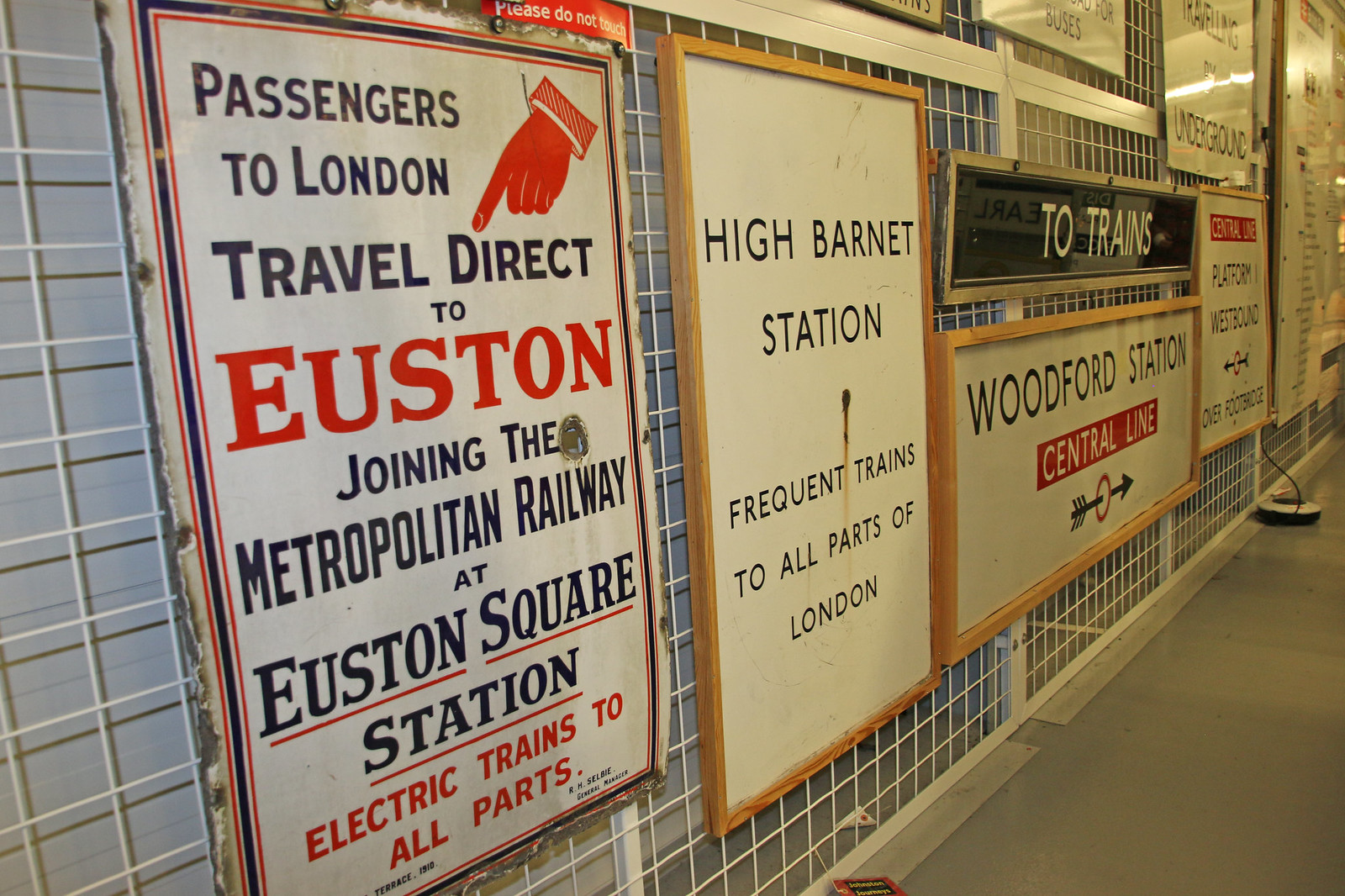The image depicts a wall with a mesh or wire background, likely situated at a London public transit station. A collection of various signs is affixed to the wall, some appearing more modern while others have an old-timey look. On the far left, a large sign framed in wood reads: "Passengers to London, travel direct to Euston, joining the Metropolitan Railway at Euston Square Station, electric trains to all parts." Next to it, another sign states: "High Barnet Station, frequent trains to all parts of London" in bold black letters on a white background. To the right, a black sign with an arrow points to "Two Trains", with "Woodford Station, Central Line" indicated below it. The signs are clearly visible in the bright overhead lighting that reflects off their surfaces, set against what seems to be a metal background behind the mesh. On the floor, there is a small round object with a coiled wire leading back into the mesh lining, adding to the intricate details of this functional yet historic station environment.